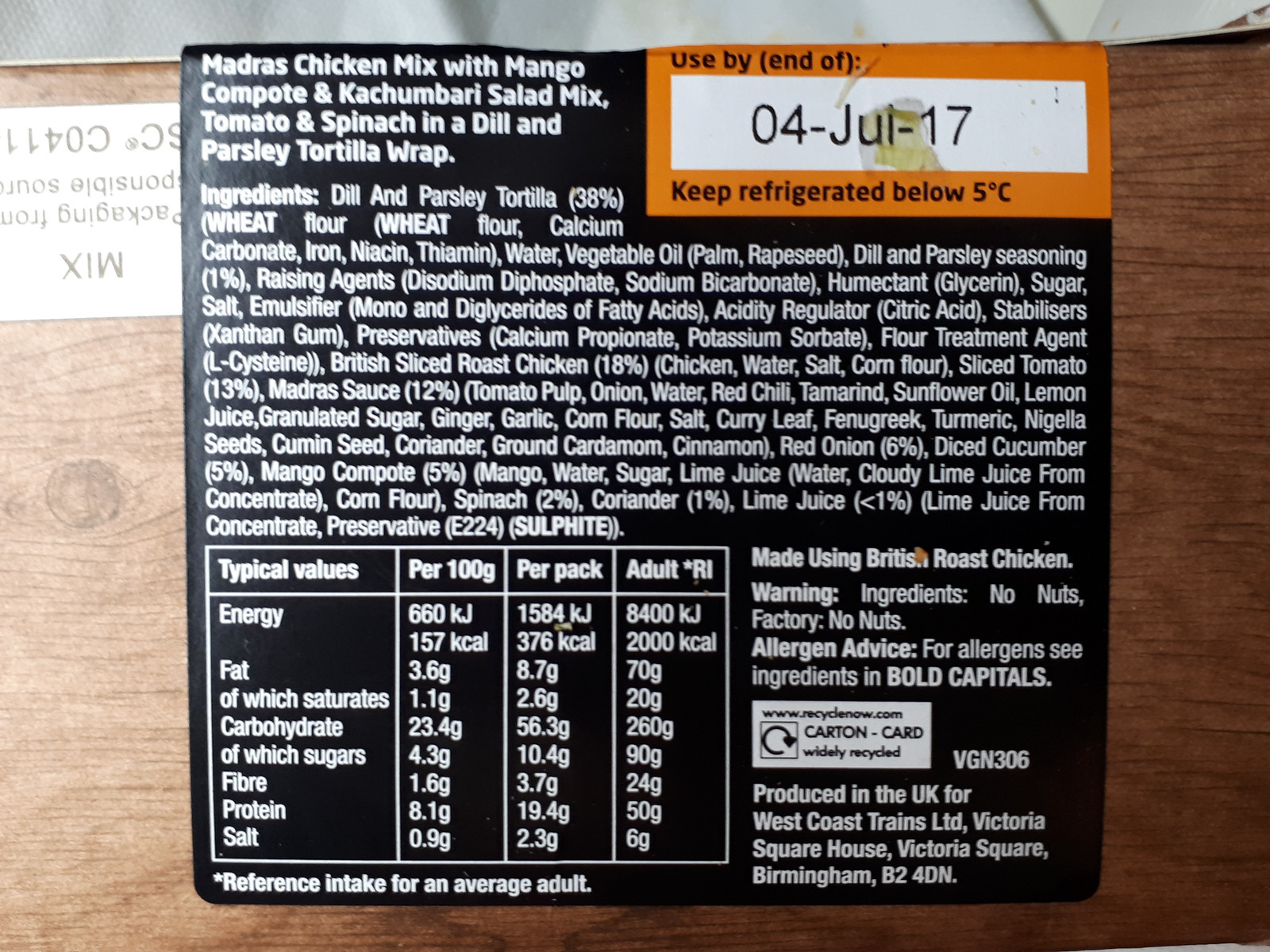This photograph features a detailed ingredient label for a Madras Chicken Mix with Mango Compote and Kachumbari Salad Mix, Tomato, and Spinach in a Dill and Parsley Tortilla Wrap. The label has a black background with white text and is placed on what appears to be a wooden table or countertop. Prominently displayed in the upper left corner is the product name, while a long list of ingredients detailing the Dill and Parsley Tortilla (38% Wheat Flour) follows. In the upper right corner, an orange rectangle with a white center indicates the use-by date as 04 July 2017, along with a note to keep the product refrigerated below 5 degrees Celsius. Below the ingredients list, nutritional information and other content details are provided. This label, distinctly British in format, hints at its production for consumers in Birmingham, United Kingdom.